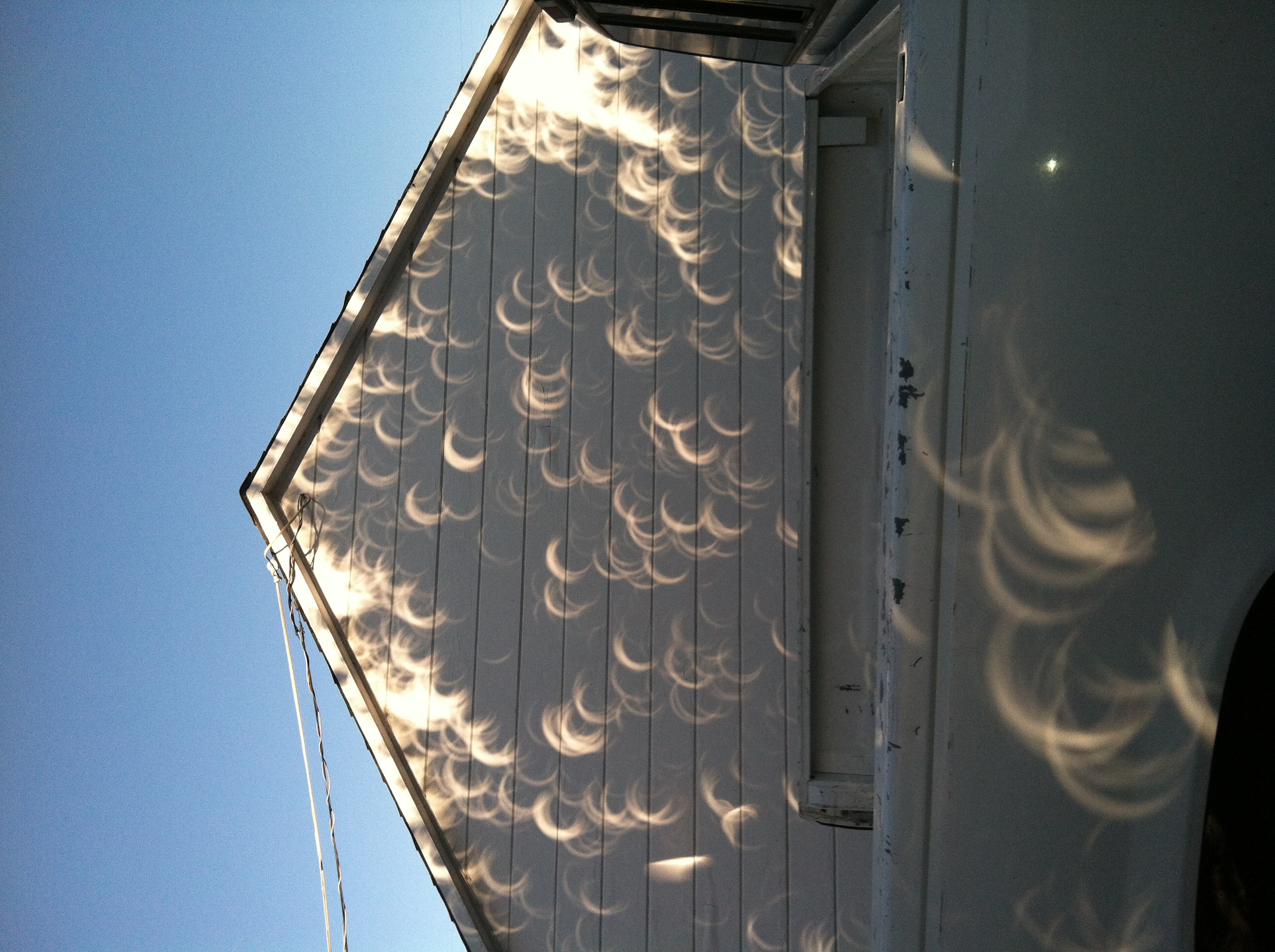The image depicts a house photographed sideways against a clear blue sky, creating the illusion of the house resting on its side. The house is painted white, with phone and cable wires extending from the crown of the roof. Sunlight bathes the side of the house, casting numerous light and dark, bubble-like shadows that resemble hallowed out circles or crescents, typically seen during a solar eclipse. These shadows scatter across the building's façade and also appear on a small matching wall in front of the house. A truck bed is also visible to the side, adding to the interesting composition of light and shadow.